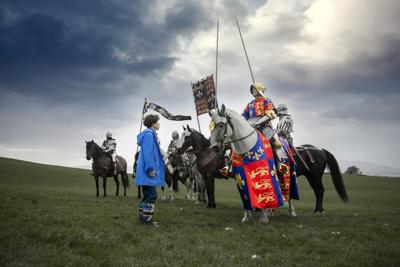The photograph captures a striking scene of a grass-covered hillside under a sky laden with heavy gray and white storm clouds. In the forefront stands a young boy, clad in a bright blue raincoat, staring intently at an armored medieval knight on a majestic white horse. The knight's attire includes a metal helmet and a tunic adorned with a gold lion on a red background, accompanied by several gold fleurs-de-lis on a dark blue backdrop. The horse sports a matching blanket and a black bridle featuring a gold plaque on its forehead. To the right, another rider in period costume holds a flag standard echoing the emblems on the knight's attire and horse blanket. Flanking the central figures are several other dark brown horses with their riders, all contributing to the medieval ambiance. The grass underfoot is lush and green, providing a vivid contrast to the darkening sky above, suggesting an impending storm from the left side of the image. The overall composition is a blend of modern and historical elements, making the scene both visually rich and intriguing.